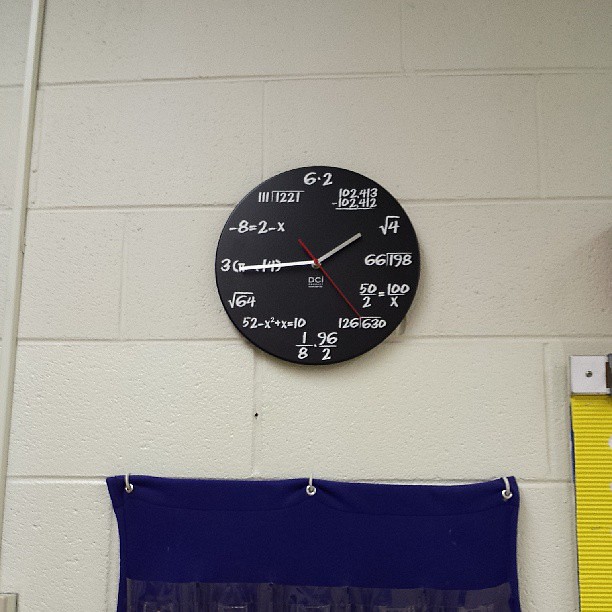This color photograph depicts a novelty black clock mounted on a white-painted brick wall. The round clock features a black background with silver hour and minute hands, and a red second hand. Uniquely, instead of regular numbers, the clock has various math problems at each hour position, written in white. For instance, at the top where 12 usually is, there is "6×2". As we move clockwise, other math problems include "1/8×96/2" at 6 o'clock, and "√4" at 2 o'clock. The clock face also has a small white logo under the hands.

The time displayed is approximately 1:45. Below the clock, a blue canvas, possibly a mat, is pinned to the wall with three hooks, featuring small round silver holes at the top and a thread coming out, suggesting it could be part of gym equipment. To the right of the blue canvas, there is a yellow object with linear details, potentially another mat or a partition placed against the wall. The setting has an academic or gymnasium-like ambiance due to the various math problems presented and the types of objects within the frame.